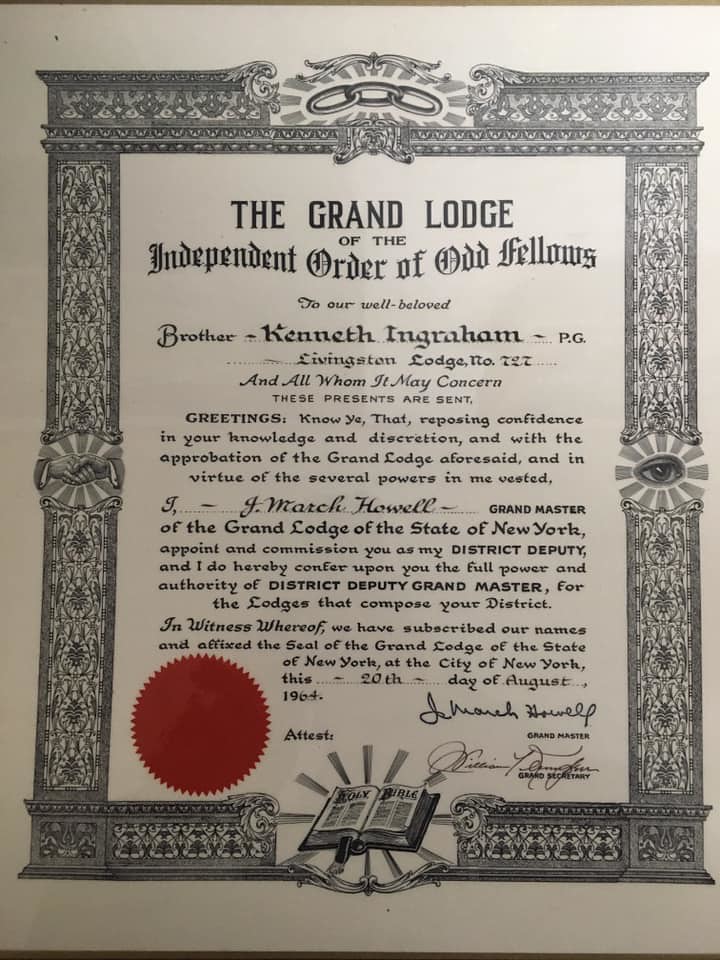The image depicts a scanned, black-and-white certificate issued by the Grand Lodge of the Independent Order of Odd Fellows. At the top, it formally acknowledges Kenneth Ingram of Livingston Lodge No. 727. The certificate announces his appointment and commissioning as District Deputy Grand Master, conferring upon him full power and authority for the lodges within his district. The document is dated August 20, 1964, and signed by J. March Howell, the Grand Master of the Grand Lodge of the State of New York. It features a gray decorative border with symbolic imagery, including eyes, a handshake, and a book. Additionally, there is a distinctive red circle with spiked edges, and several signatures are present at the bottom right. The background of the certificate is light gray, with text written in black.